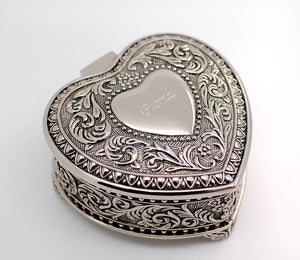This photograph captures a detailed, antique silver jewelry box in the shape of a heart. The box is ornately decorated with intricate filigree patterns, etched leaves, and small flowers distributed across its surface. At the very center of the lid is a smooth, unembellished heart, engraved with the name "Fiona" in a script that appears somewhat faded. This central heart features a reflective, glass-like or mirror-like surface. The jewelry box, which opens from the front and hinges at the back where the heart dips down, stands on small feet adorned with additional filigree. The entire piece rests on a white surface, casting a subtle shadow on the lower left side of the image, accentuating its elegant contours and exquisite craftsmanship.